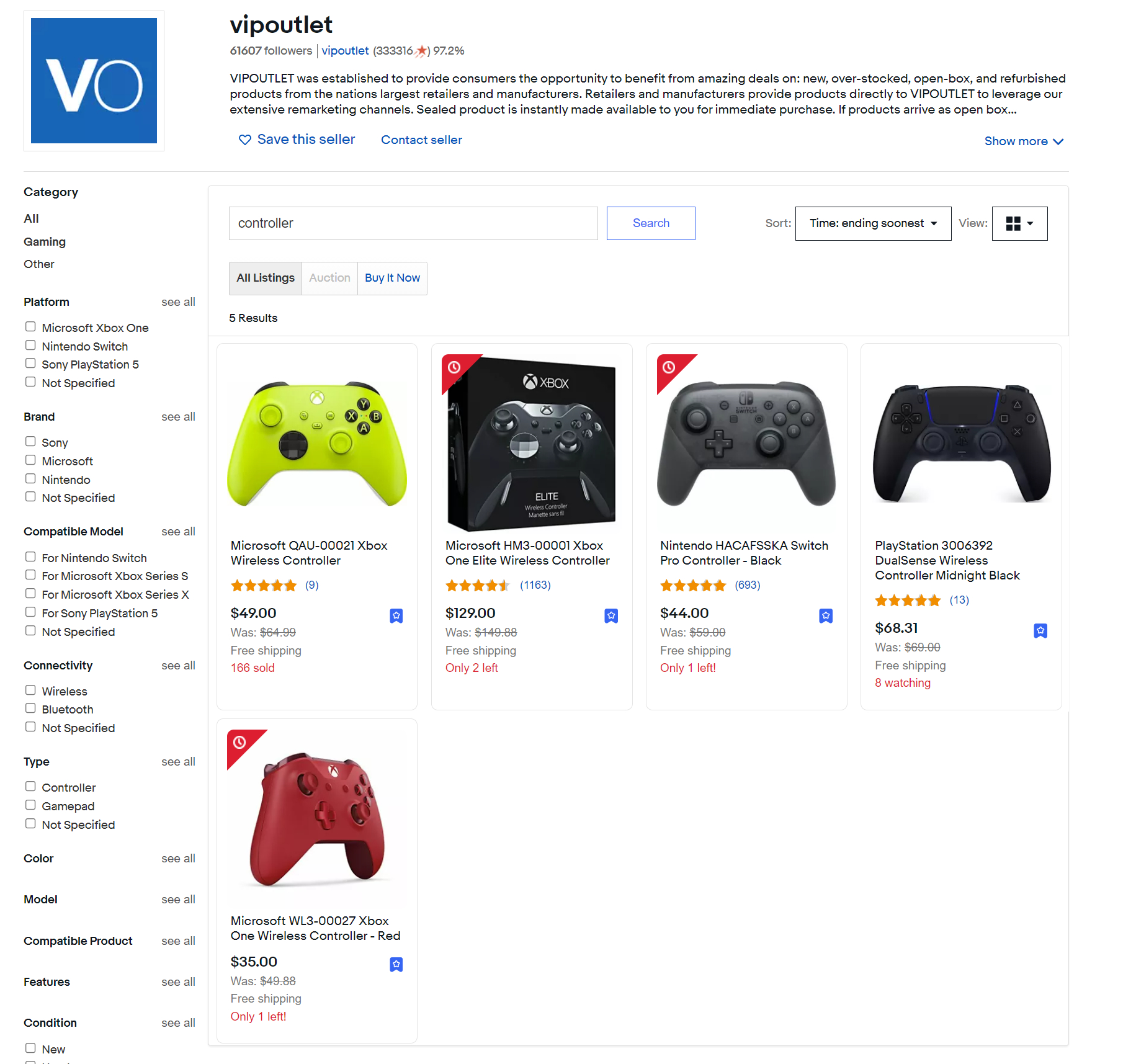This is an image from the website VIP Outlet. In the upper left-hand corner, there is a logo for VIP Outlet, which consists of a blue square featuring a stylized white letter "V" and a thinner white letter "O" beside it. To the right of the logo, "VIP Outlet" is displayed prominently, indicating the name of the site. The site boasts a follower count of 61,607, which is shown below its name.

Beneath this header, a section dedicated to controllers is showcased, listing five different results. The first item displayed is a yellow Microsoft controller. Following that is a more detailed listing: the Microsoft HM30000 Xbox One Elite Wireless Controller. Continuing down, the third controller is identified as the Nintendo Switch Pro Controller. The fourth item in the collection is a PlayStation controller, unspecified in detail. Finally, at the bottom of the list, there is another Microsoft controller, the XL3 model.